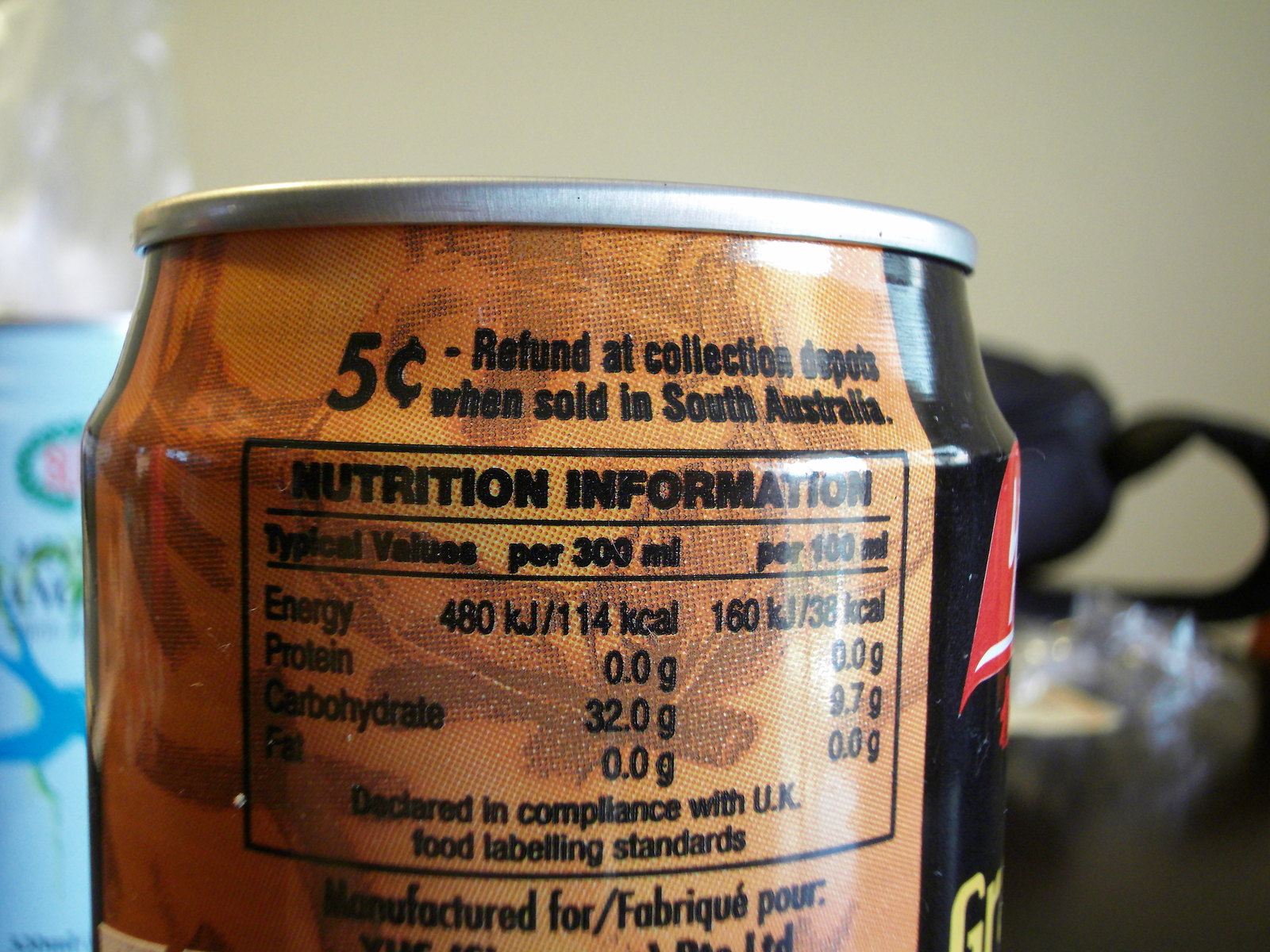This image showcases a close-up of the side of a can. The can prominently displays a statement indicating that it offers a 5-cent refund at collection depots when sold in South Australia. The primary focus of the image is on the nutritional information, which details the content of energy, carbohydrates, protein, and calories, expressed in kilojoules for a 300ml serving. It is also noted that the can complies with UK food labeling standards. The main label, including the product type, logo, and company name, is not visible in this image. The visible portion of the can is predominantly black, featuring a red front section. The background is slightly blurred, revealing a table on which a bag and possibly another can are situated next to the can in the center of the image.